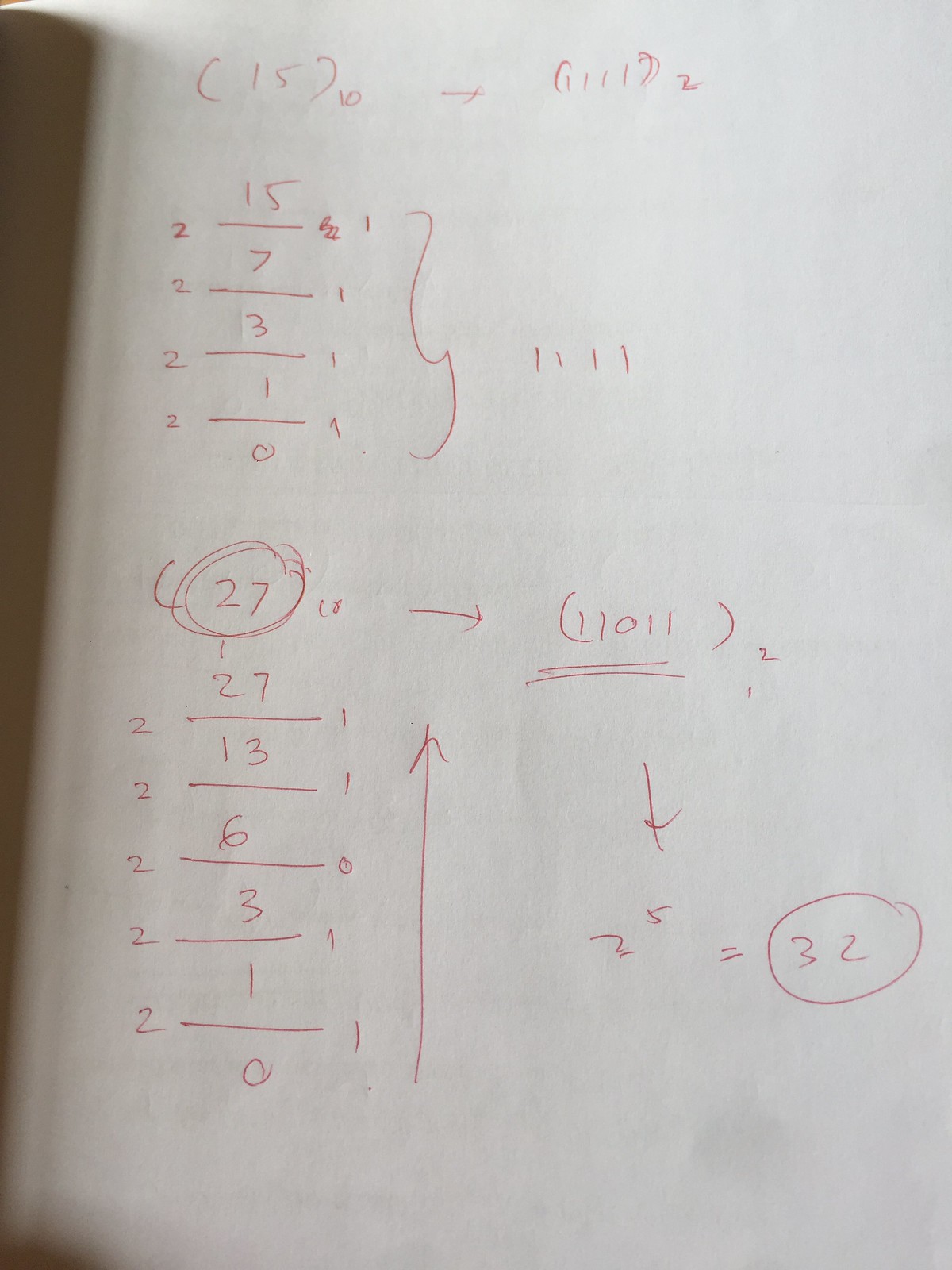This image depicts a piece of paper densely covered in red numerical writing, primarily consisting of equations and fractions. 

At the very top of the page, there is an expression beginning with parentheses containing the number 15. Adjacent to this, on the lower right-hand side but outside the parentheses, is the number 10. This is followed by a minus sign and another parenthetical expression containing the number 1111 (one thousand one hundred and eleven), with the number 2 positioned on the lower right-hand side just outside these parentheses.

Beneath this, there is a sequence of fractions vertically aligned: 
- The number 2 followed by 15/7,
- The number 2 followed by 7/3,
- The number 2 followed by 3/1,
- The number 2 followed by 1/0.

Separating these numerals from the next section is a squiggly line. To the right of this line, the sequence '1111' (one thousand one hundred and eleven) appears prominently.

Below this is another line, under which the number 27 is written, accompanied by an arrow pointing towards the number 11011 enclosed in parentheses, with a small number 2 positioned to the upper right-hand corner of the parentheses.

Following this, a new set of fractions is written, again vertically stacked:
- The number 2 followed by 27/13,
- The number 2 followed by 13/6,
- The number 2 followed by 6/3,
- The number 2 followed by 3/1,
- The number 2 followed by 1/0.

On the lower right-hand side of these fractions, there seems to be a notation with the number 2, and an additional smaller 5 in the upper right corner, which equals 32.

This paper appears to be filled with complex mathematical operations and notations, potentially indicating advanced problem-solving work.